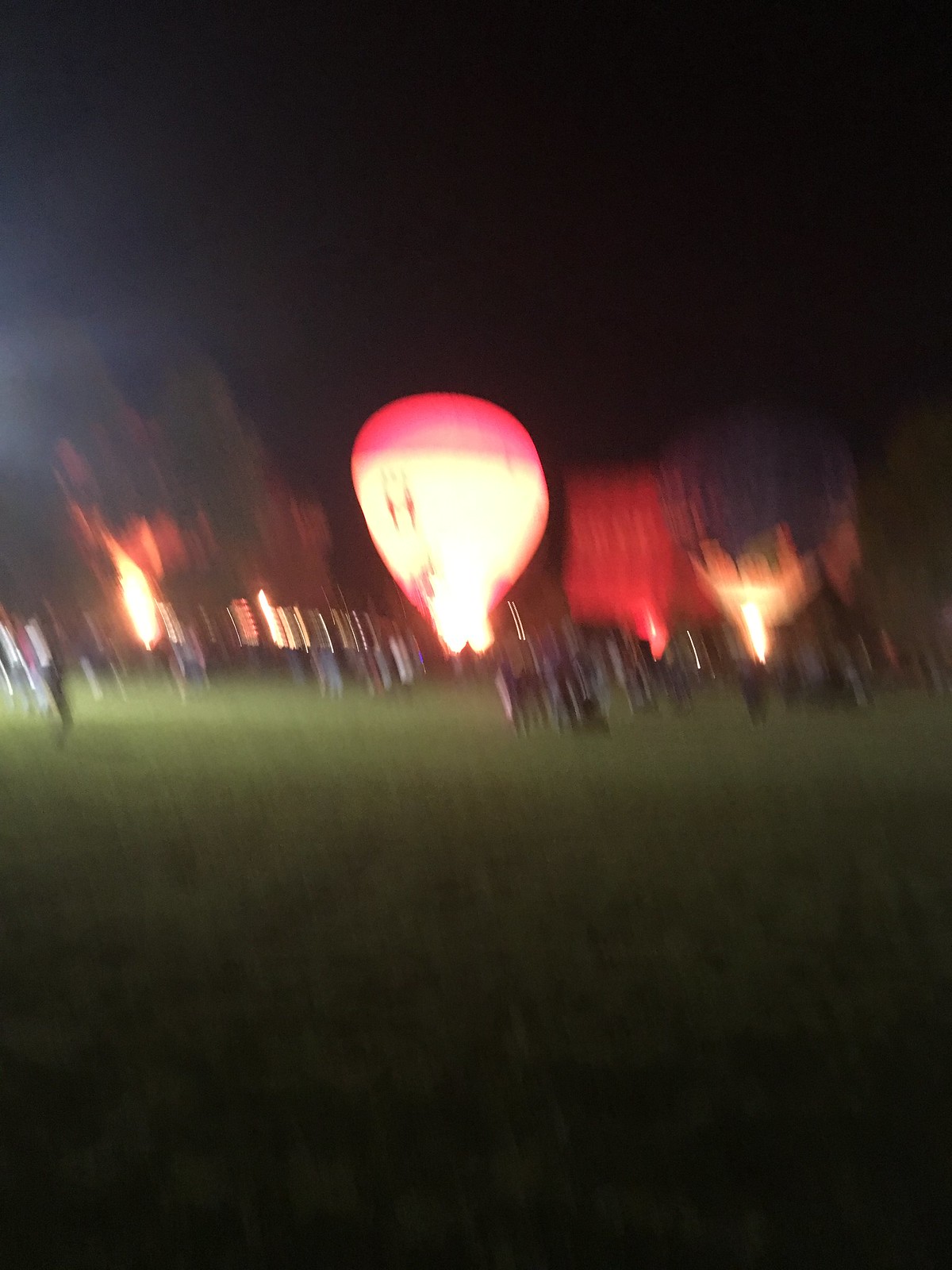In this nighttime photograph, a fleet of aerial balloons is poised for takeoff on a low-cut, grassy field. The scene is somewhat blurry, lending a dreamy quality to the image. Large crowds of onlookers are visible in the distance, adding to the sense of anticipation. The balloons are partially illuminated by the glow of ignited gas, casting a warm light over the scene. Dominating the center is a balloon with a white lower section and striking red top. Adjacent to it is a dark blue balloon, contrasting against the night sky. The horizon is framed by silhouetted trees on either side, completing the composition with a serene, natural border.